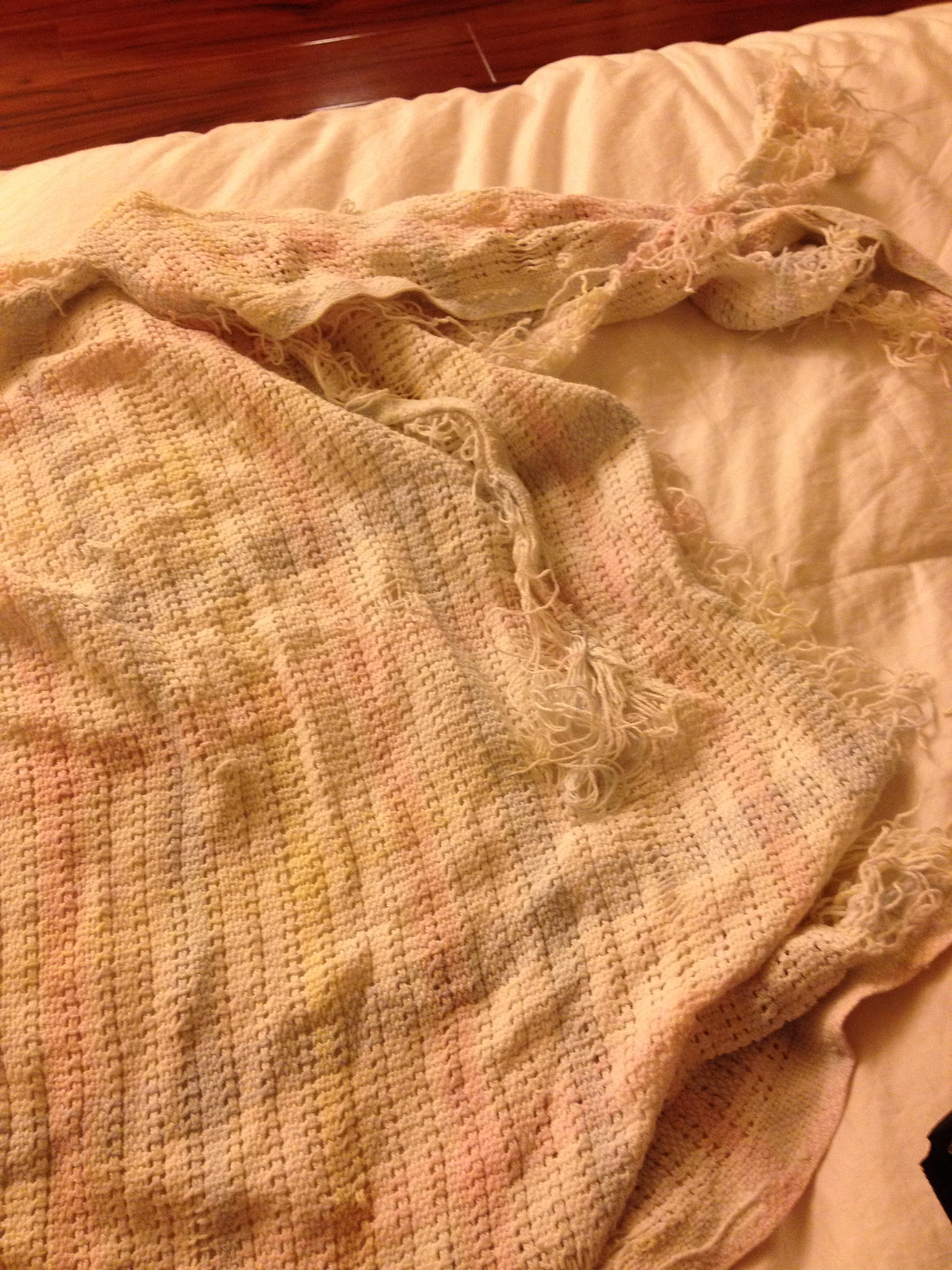This detailed photograph depicts a double-sized bed featuring a torn, hand-knitted quilted blanket with a cream base interspersed with very faded streaks of pink, yellow, and faint hints of red and blue. The blanket prominently occupies the majority of the image and is torn along the upper middle right, with threads visibly fraying and some sections twisted up. The bed is made up with wrinkled white sheets underneath the blanket and no visible pillows or cover. A portion of rich, reddish-brown wooden floor planks can be seen in the upper left corner of the image, adding a touch of contrast. No people or discernible objects, apart from some indistinct black item at the bottom right, appear in the photograph. The intimate, cozy setting and the damaged yet endearing blanket dominate the serene composition.